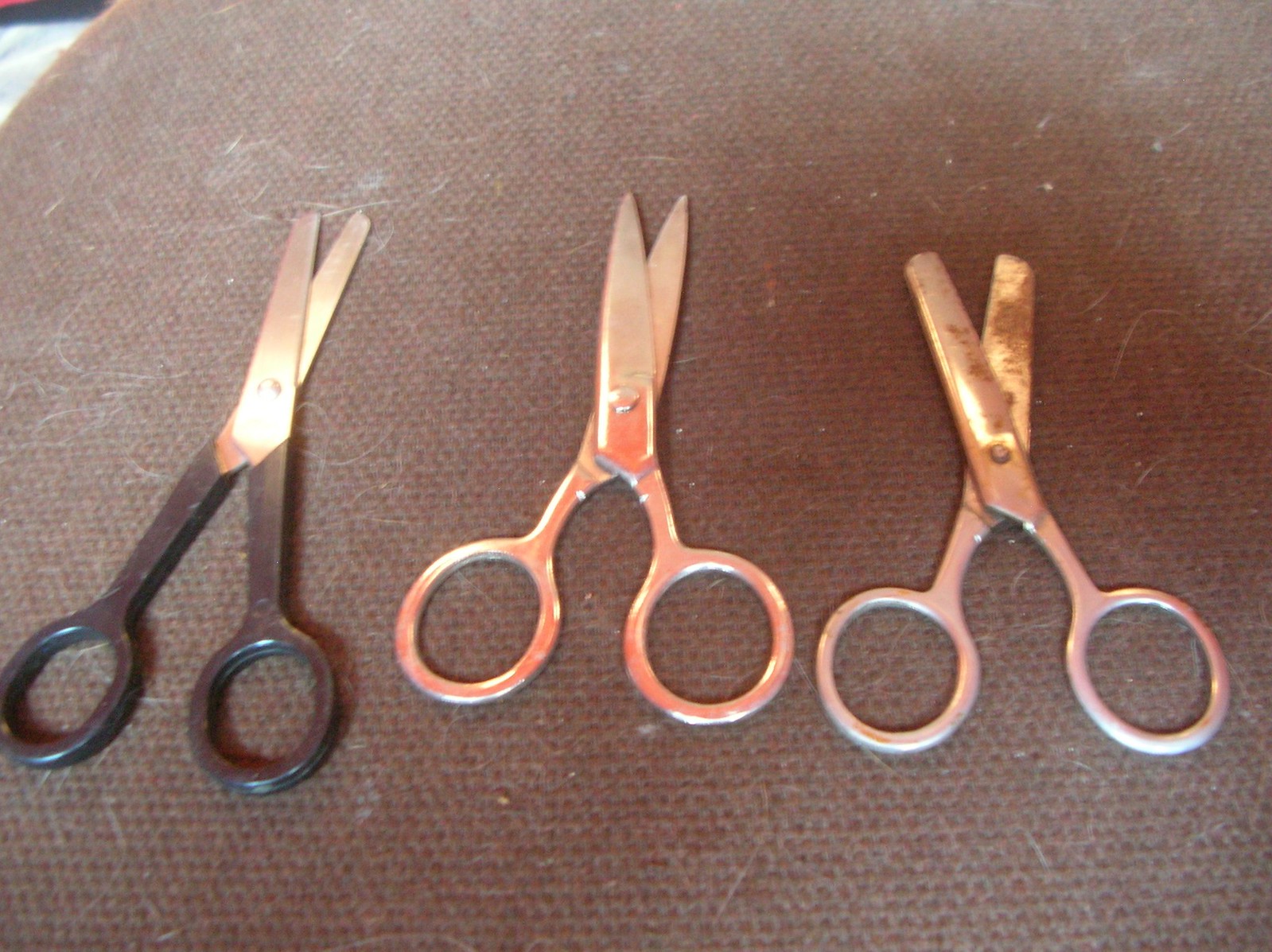This image is a close-up photograph of three pairs of scissors lined up side by side on a fabric surface. The fabric is brown and covered with numerous light-colored hairs, possibly from an animal like a white cat. The scissors are arranged with their handles at the bottom and their blades pointing upward, each pair slightly open at the same angle. 

The first pair of scissors on the left features stainless steel blades and black-painted handles, appearing taller and skinnier than the others. The middle pair is entirely made of stainless steel with sharp, angled blade tips. The third pair on the right is also stainless steel but has rounded, blunt tips and appears slightly rusty, resembling safety scissors. This detailed layout highlights the variations in design and condition among the three pairs of scissors against a hair-covered fabric backdrop.